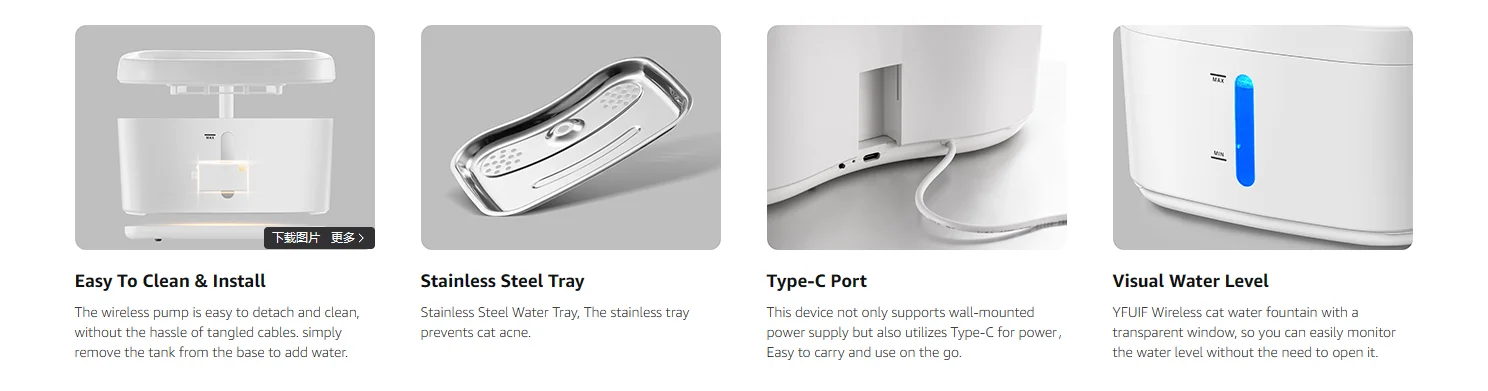The image showcases a four-step guide to using a wireless cat water fountain, each step represented by a photograph on a medium gray background arranged in a row from left to right against a white backdrop. 

1. The first photograph highlights the wireless pump with the caption, "Easy to Clean and Install." It emphasizes that the pump is easy to detach and clean without the hassle of tangled cables. The image shows the pump being removed from the base, indicating how simple it is to add water by removing the tank.

2. The second photograph features a diagonal stainless steel tray in the center, accompanied by the caption, "Stainless Steel Water Tray." This stainless steel tray is designed to prevent cat acne, ensuring a healthier drinking environment for pets.

3. The third photograph focuses on the device's power port, displaying a Type-C connector with a cord plugged into a sleek white electronic piece of equipment. The caption, "Type-C Port," explains that the device not only supports wall-mounted power supply but also utilizes a Type-C port for easy portability and use on the go.

4. The last photograph to the right illustrates a bright blue water line within a transparent water fountain window and is captioned, "Visual Water Level." It describes how the YFUIF wireless cat water fountain has a transparent window that allows users to monitor the water level effortlessly without needing to open the unit.